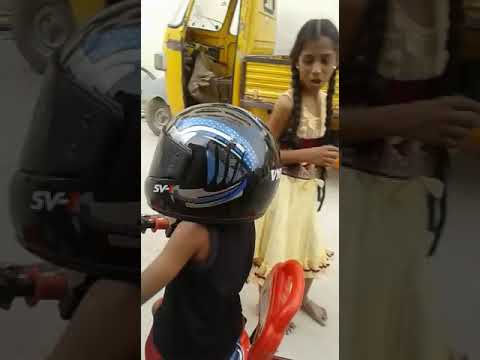The image is a detailed, three-panel composition. The central panel, which is slightly larger than its flanking counterparts, features a small, dark-skinned child riding a tricycle with training wheels. The child is captured from behind, moving up and to the left on a gray cement surface. The child wears a black helmet emblazoned with white letters that might read "DNC," "BNC," or "VMG." A black shirt, red shorts, and possibly tennis shoes complete the outfit. The tricycle sports a red seat and has a small red rack extending from the back.

The background includes a light pale yellow wall with a bucket on a ledge, a tree or green branches growing up the side of the wall, and an adult bicycle propped against the wall. A long coil, likely a hose, can be seen in the vicinity. 

The left panel is a darker, close-up shot of the child's left side, highlighting the left arm, hand, and leg while cutting off at the torso. The right panel is also darkened, showing only the cement ground and a partial view of the adult bicycle’s wheel at the top edge. This framing with darkened and enlarged sections of the central image provides a cohesive border around the main scene.